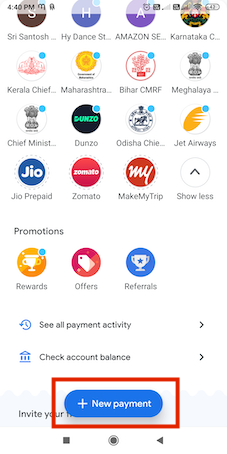A screenshot of a smartphone screen at 4:40 PM, showcasing various app icons and notifications. The visible app icons include Siri Santosh, iDance ST, Amazon SE, Karnataka SE, Kerala Chef, Maharashtra, Bihar, Meghalaya, Chef Ministry, Dunzo, Odisha Chef, Jet Airways, Jio Prepaid, Zomato, and Make My Trip. Each app is represented by its unique icon, contributing to the colorful and cluttered display.

In the middle of the screen, there's a prominent section with the heading "Show Less," which suggests the presence of additional promotional content that can be minimized. This section includes options like Rewards, Offers, and Referrals. Another noticeable feature is the "All Payment Activity" area, which includes options like Check Account Balance.

A highlighted notification in blue with a red outline indicates a new payment form, suggesting the user is prompted to make a payment, potentially to one of the frequently used apps indicated on the screen. The red background adds a distinct contrast, making this notification stand out in the otherwise busy interface.